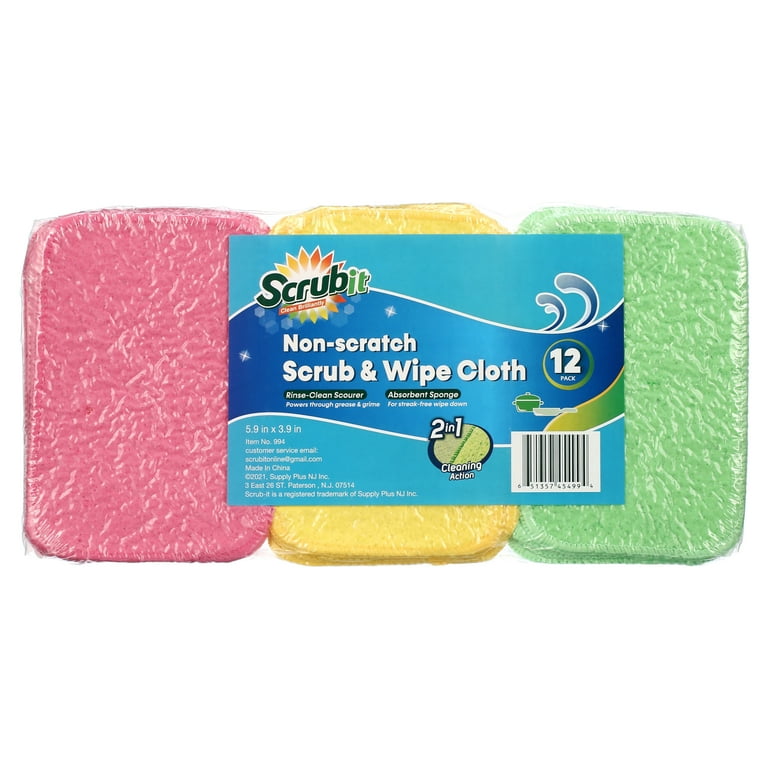The product image features a 12-pack of "Scrub It" non-scratch scrub and wipe cloths, prominently displaying three sponges in pink, yellow, and green from left to right. Each sponge is individually vacuum-sealed in shrink wrap, preserving their form and cleanliness. The package is topped with a vibrant green label adorned with a blue wave design, which showcases critical product details: "Scrub It" non-scratch scrub and wipe cloth, 12-pack, rinse clean, scourer, absorbent sponge, 2-in-1 cleaning action. The dimensions of each sponge are clearly listed as 5.9 inches by 3.9 inches, and the item is identified by the item number 994. Manufactured in China, the package also features a barcode located on the bottom right corner, ensuring easy scanning. The entire package is set against a plain white background, making the colorful sponges and detailed labeling stand out.